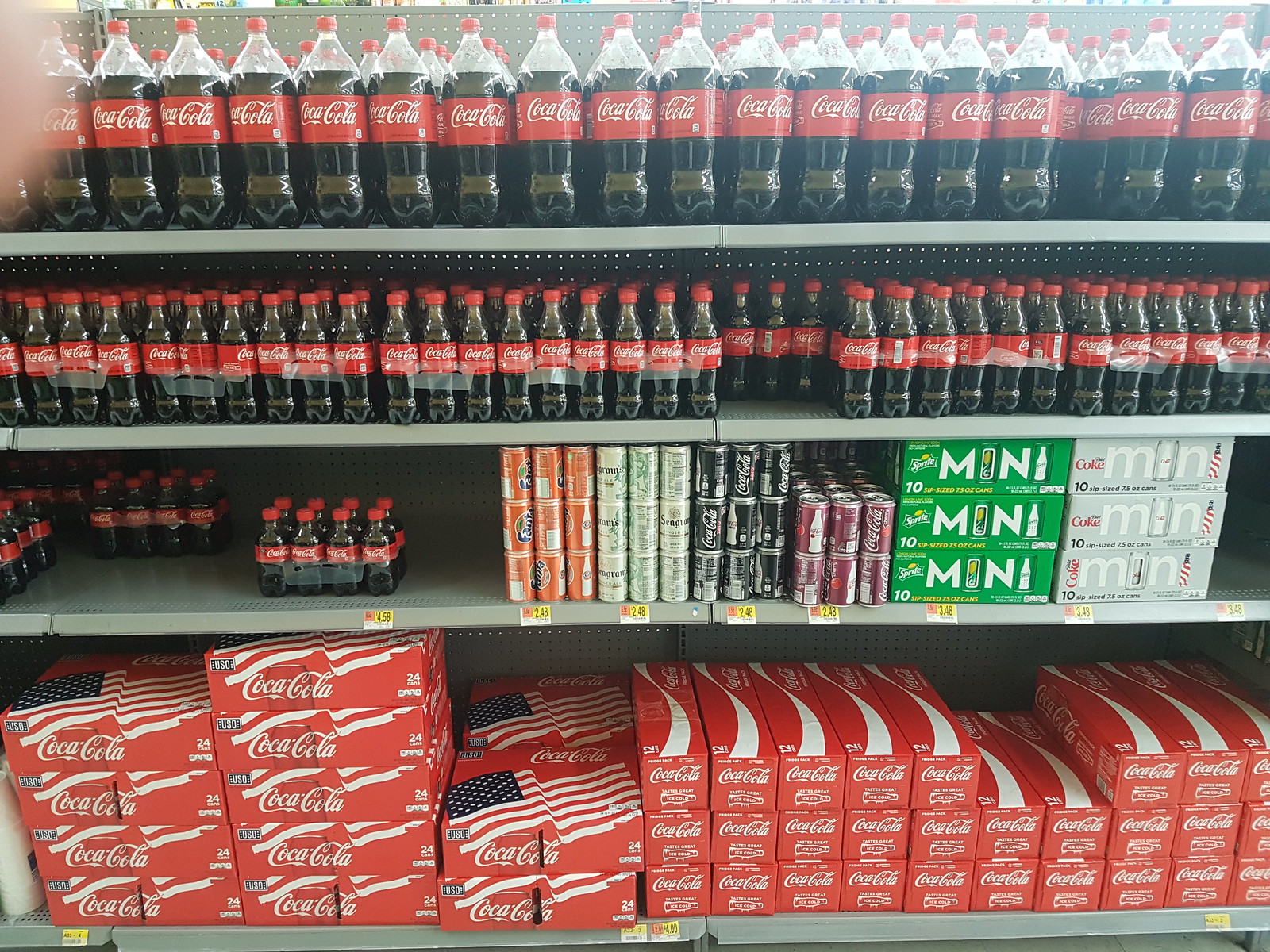The photograph captures a well-organized display of Coca-Cola products on grocery store shelves. The shelving unit consists of four gray shelves adorned with yellow price tags, indicating prices that range from $2.48 to $4.58 for various products. The top shelf showcases one-liter or two-liter bottles of Coca-Cola, easily recognizable by their brown soda and iconic red labels with white Coca-Cola lettering. The second shelf features six-packs of 20-ounce Coca-Cola bottles. The third shelf down houses smaller, eight-pack miniature bottles of Coca-Cola alongside an assortment of miniature cans, including Fanta, Seagram's, Coke Zero, Coke Cherry, mini Sprite, and mini Diet Coke. The bottom shelf is stocked with Coca-Cola products in larger quantities: 12-packs in distinctive red and white boxes occupy the bottom right corner, while 24-packs, adorned with an American flag on the top, add a patriotic touch to the display.